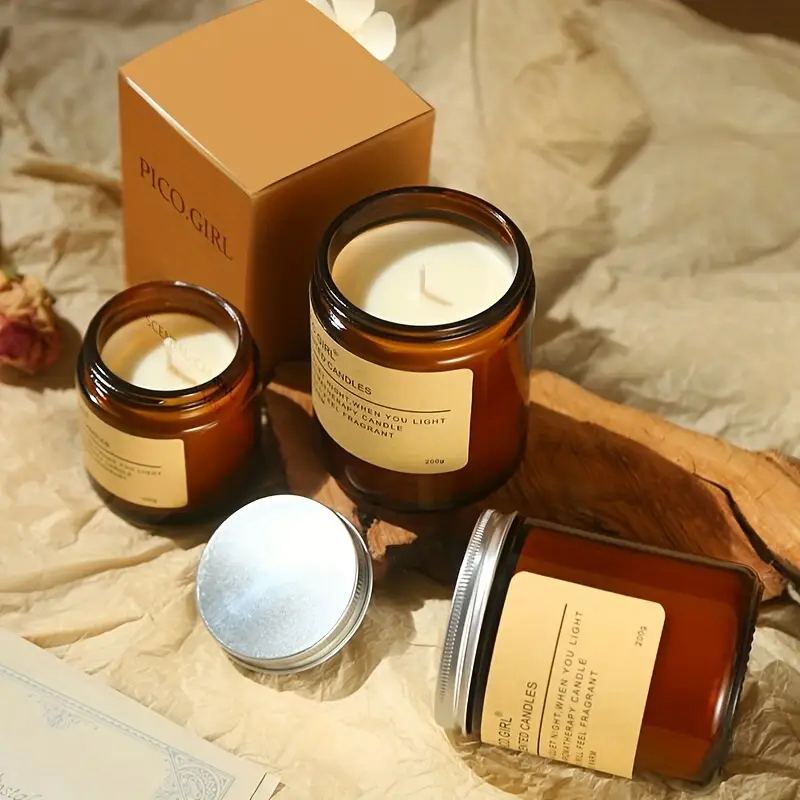The photograph features an assortment of elegant white wax candles encased in brown glass jars with tan labels, creating a sophisticated display. Each jar, labeled with the name "Pico Girl," is distinguished by its rustic and aesthetic design elements. One jar lies on its side with a metal lid, while another rests in a wooden, rustic-looking candle holder. Surrounding the candles are delicate flower petals and scattered papers, all set on a light brown, possibly cloth or paper, background. A tan-colored box prominently displaying the name "Pico Girl" accentuates the scene, hinting at the refined packaging of these presumably scented aromatherapy candles. The top-down shot provides a comprehensive view, highlighting the elegant arrangement and the inviting ambiance these candles create.